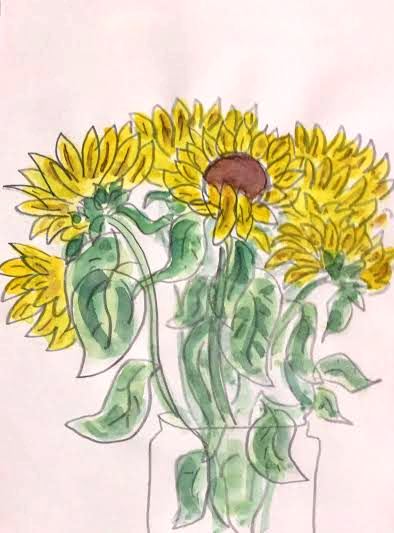This is a detailed crayon drawing of sunflowers in a glass vase, set against a pale pink background. There are seven sunflowers in total, each adorned with vibrant yellow petals featuring darker yellow-brown lines, giving them texture and depth. The outline of the vase and the flowers appears to be drawn in pencil or a single crayon line, lending an understated, simple elegance to the composition. Each sunflower has long green stems with numerous leaves, and the flowers are uniformly sized but face different directions, creating a dynamic sense of movement. Only one sunflower prominently displays its brown center, making it a focal point amidst the uniformly yellow blooms. The arrangement of the flowers in the vase, with petals varying slightly in formation—some perfectly aligned and others more misshapen—adds to the natural, lifelike quality of the artwork.